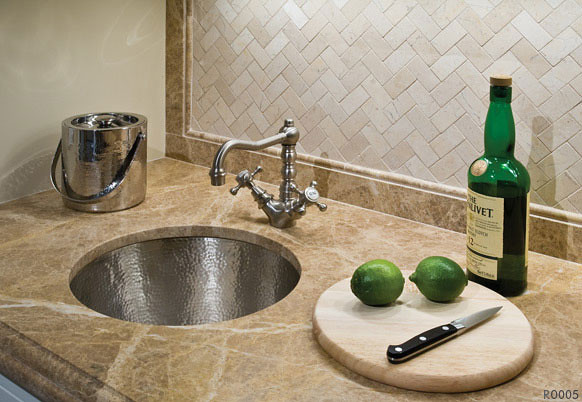This photograph, labeled "R0005" in black font at the bottom, captures an elegant wet bar setup. The focal point is a tan and gray stone backsplash that is bordered by a marbled edge in shades of tan and brown. On the countertop, a green bottle with a brown cork and white label casts a shadow against the backsplash. In front of the bottle lies a pale off-white cutting board with two limes on it. A silver knife with a black handle rests nearby. 

The wet bar features a sleek silver faucet and a matching sink basin. To the other side of the sink, there is a silver ice bucket with a silver handle. The countertop itself is adorned with a white marbled surface featuring splashes of brown, tan, and white, which complements the glimpse of white cabinetry beneath it. This detailed arrangement offers a luxurious and inviting atmosphere.